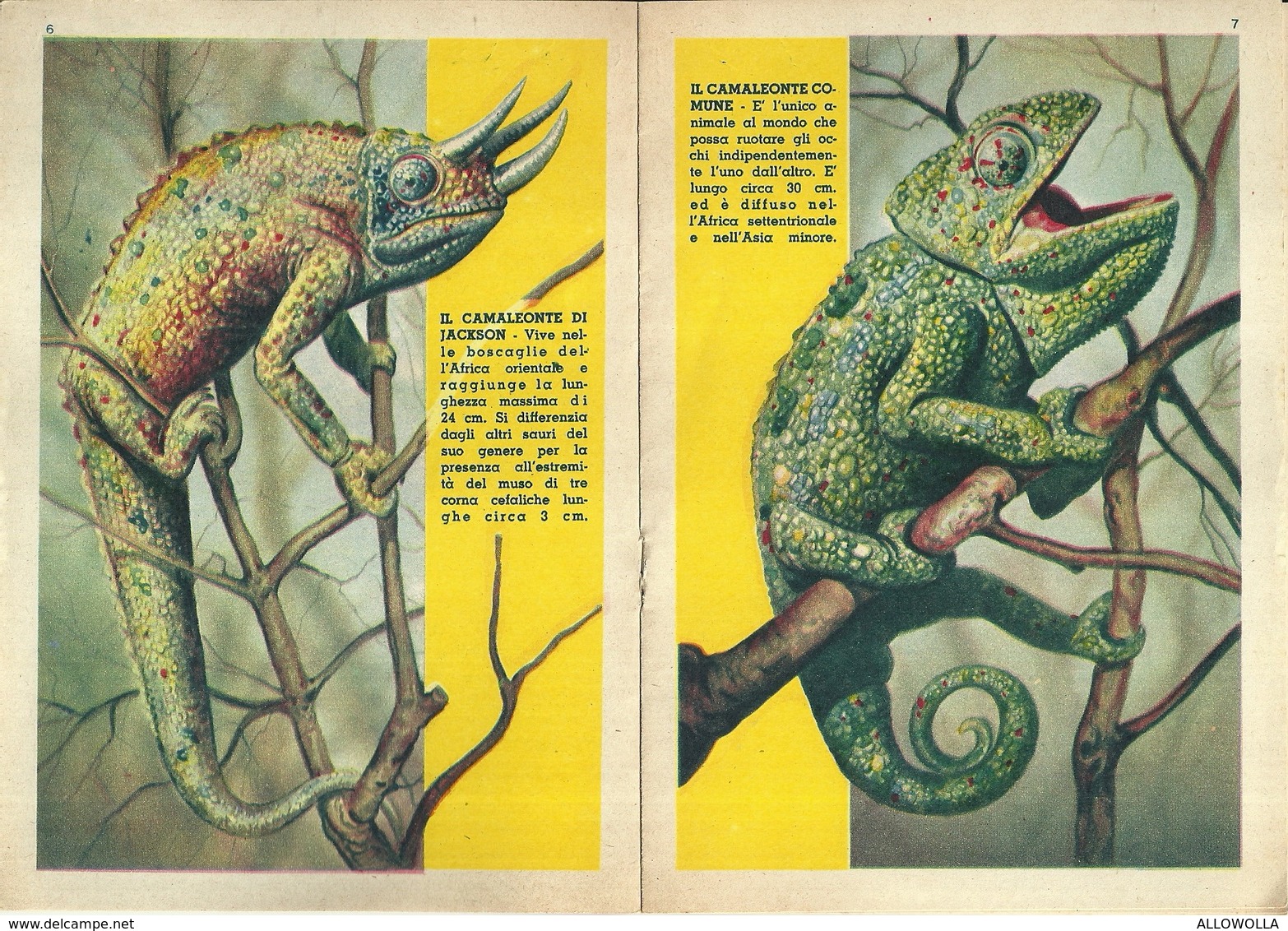The image depicts two scanned pages from an old textbook or magazine focusing on wildlife, specifically chameleons. The left page, numbered "6," features a three-horned chameleon, also known as Jackson's chameleon, clinging to a tree branch with its claws and tail for support. Its vibrant coloration includes shades of green, gray, red, yellow, and orange. The text beside it, written in Italian within a yellow bar, describes the chameleon’s habitat in East Africa and distinctive three horns on its head. On the right page, numbered "7," another chameleon is depicted with its mouth open, revealing a red tongue, and its tail curled into a spiral. This chameleon is adorned with green, blue, red, and yellow spots, with noticeable red around its eyes and restricted, scaly skin protecting them. The accompanying text, also in an Italian yellow bar, explains the ability of this common chameleon to move its eyes independently. The URL www.delcampe.net appears at the bottom left corner of the left page, and the name "Alawalo" or similar is written on the bottom right corner of the right page.